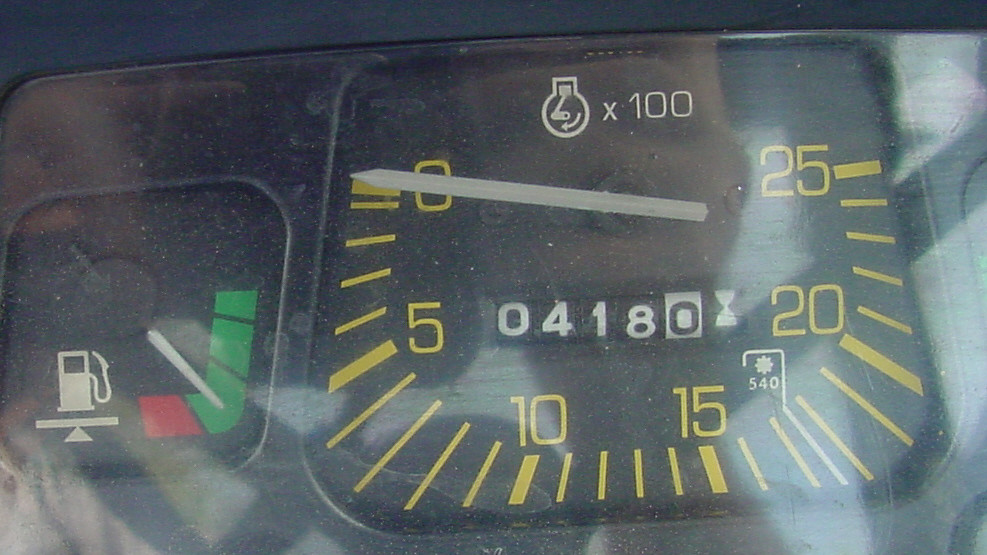This photograph captures a close-up view of a vehicle's dashboard instrument panel, with a glossy reflection of sunlight visible across the surface. On the left side of the panel, there is an icon that resembles a gas pump, indicative of the fuel gauge. Within this circle, there is a white needle indicating the fuel level. Adjacent to the gas pump icon, there is a red square symbol followed by a green strip, likely representing warning or status indicators.

On the right side of the dashboard, an abstract circular icon is displayed, featuring an "X" and the number "100" in yellow font. Surrounding this icon is a semi-circular arrangement of yellow numbers, marked in 5-unit increments starting from 0 up to 25, accompanied by yellow dash marks between each number. In the center of the instrument panel, a digital display shows the numbers "0418" in white and black font, while the number "0" is highlighted in black. The combination of these elements provides essential information about the vehicle's status and operational metrics.